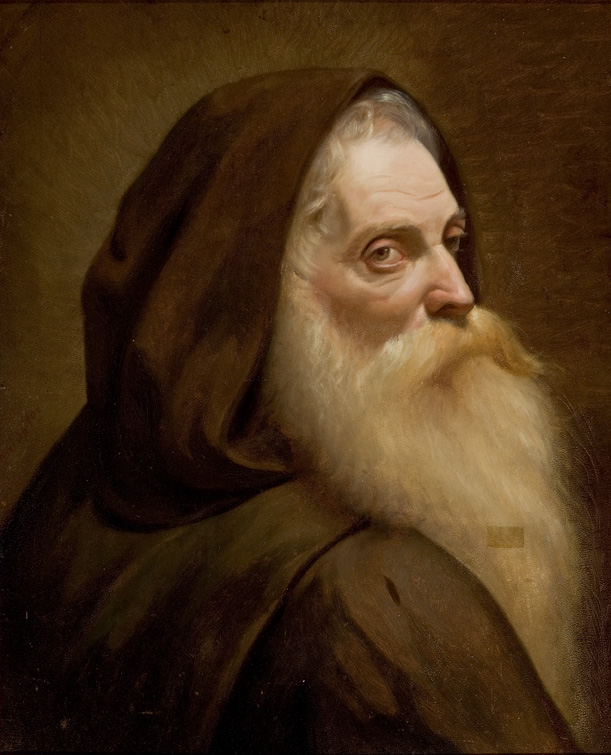This painting features an older man, depicted in a highly realistic and detailed style, suggestive of Renaissance or Impressionist influences. The subject is a white-skinned gentleman with a long, flowing white beard that contains hints of blond, particularly around the mustache, giving it a slightly yellowed appearance. He appears serious and contemplative, his sad, deep-set eyes gazing out toward the front from the right side. His detailed, weathered face with intricate wrinkles speaks to his advanced age.

Clad in a dramatic, flowing red robe and hood that covers his head, the man exudes a solemn, almost religious presence. The artwork hints at a dramatic light source from behind the subject, casting the surrounding area in a golden-beige hue that gradually darkens at the edges. The background itself is predominantly brown, adding to the painting's rich, subdued tones.

Overall, the artistry captures an intense realism through the well-blended skin tones, meticulously rendered facial features, and the textured beard, emphasizing the man's venerable and austere appearance against the minimalist backdrop.